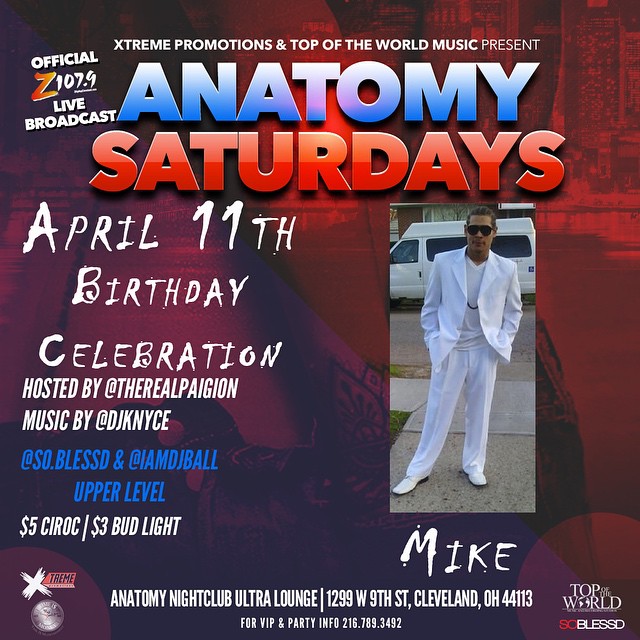This image appears to be a detailed promotional flyer for an event called "Anatomy Saturdays." The flyer has a background that transitions from red in the upper right corner to purple in the lower left. The backdrop seems to suggest a city street with buildings and a railing, possibly featuring a person's arm against the purple area.

Dominating the center of the flyer is a vertical rectangular image of a handsome man in his twenties, dressed in an eye-catching, almost 80s-style outfit. He wears a white v-neck t-shirt, a white suit jacket, flowy white pants, and black aviator sunglasses. The man stands confidently on a sidewalk, with a somewhat shabby van parked behind him. Below his image, the name "Mike" is printed in white.

At the top of the square flyer, bold text reads "Anatomy Saturdays," with "Anatomy" in light blue and "Saturdays" in orange. Additional details reveal that it's an "April 11th Birthday Celebration," with specifics on hosts and musicians: "Hosted by @TheRealAlpagian, Music by @DJKNice, @So.Blessed, and @IAmDJBall," the latter two labeled as "upper level." Drink specials are also advertised with "$5 Siroc" and "$3 Bud Light." The flyer is further branded with “Extreme Promotions and Top of the World Music” and mentions an “official Z107.9 live broadcast.” The event's location is given as "Anatomy Nightclub Ultra Lounge, 1299 West 9th Street, Cleveland, Ohio 44113," and there are various logos scattered throughout.

Overall, the flyer is a vibrant and visually compelling invite to a special event with music, drinks, and a stylish setting.